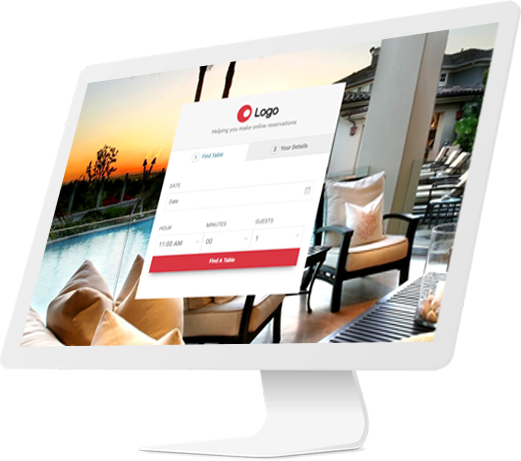The image is an advertisement displaying what appears to be a digitally rendered desktop computer. On the screen of the computer, there is an image showcasing a luxurious vacation property. The foreground features a serene poolside seating area with stylish black chairs adorned with off-white pillows, and an off-white table that has a decorative glass container filled with seashells. Additional chairs can be seen to the side, along with a tan column adding to the elegant setting.

The background of the image is bathed in a beautiful orange and yellow sunset, enhancing the tropical ambiance. Illuminated tiki torches add a warm, inviting glow. The setting includes a sparkling pool and a tree, situated near a house with a dark-colored roof.

In the center of the screen, there is a gray box displaying placeholder text—where the company name and logo should be—depicted with the words "Company Name" in black and a red circle with a smaller white circle inside it next to the text. Below it, a sentence of black text is partially visible. Further below, blue font and several selection fields allow users to choose dates, hours, minutes, and guests, accompanied by a red and white button for submission. The top menu area features the words "Your Details" in barely readable, blurry font, indicating a form or reservation system.

Beyond these elements, there are no additional visual details of note in the image.